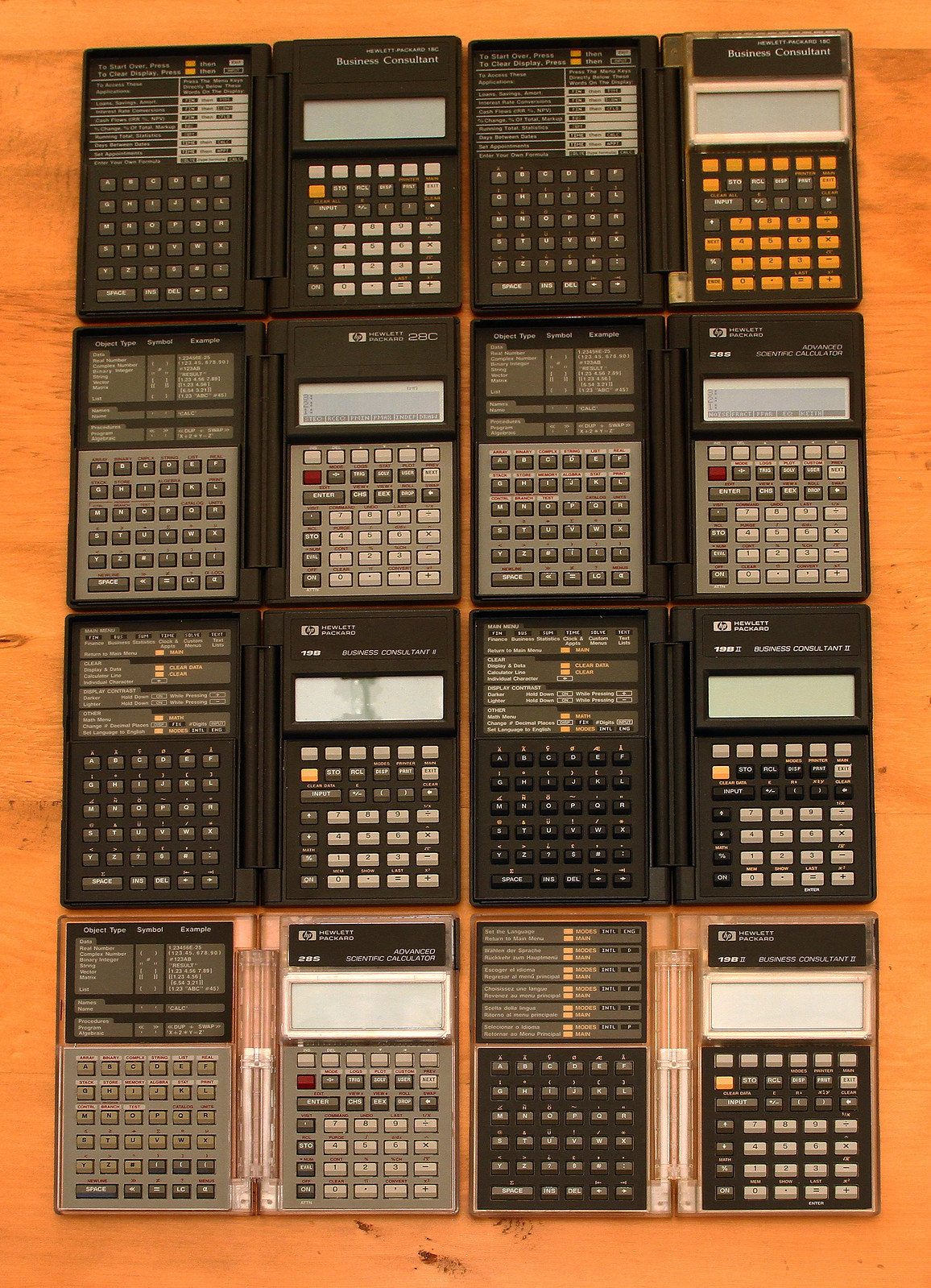This image features a collection of various electronic devices that resemble calculators but have multiple functionalities, extending beyond just number input. These devices are meticulously arranged on a light wooden table in a 4x4 grid, suggesting a total of 16 units. They share a general structure, appearing to have a left side with alphabetic keys and a right side with typical calculator keys, implying that they can fold shut like mini laptops. The color palette of the devices predominantly includes blacks, grays, and dark grays, with several featuring orange, yellow, off-pink, and white accents. Notably, some devices have large screens at the top while others have smaller ones, displaying a mix of writings, blank screens, and images—one even resembling a tornado. Certain buttons are highlighted with reds, oranges, and whites, and a brand, 'HP,' along with text like 'business consultant,' is visible on some devices, indicating they are sophisticated calculators or organizational tools rather than simple numeric calculators.